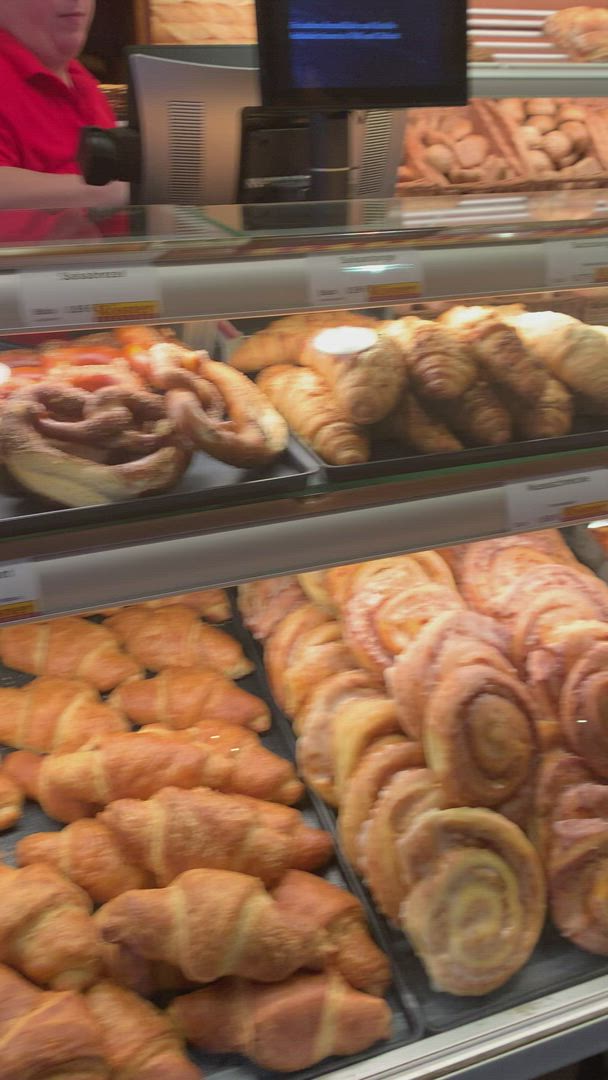This close-up photograph, taken inside a bakery, showcases an assortment of baked goods neatly arranged on shelves. At the bottom shelf, there's a large tray filled with golden-brown croissants and an assortment of round pastries, some of which appear to be cinnamon rolls, suggesting they might have a filling. Adjacent to these, on the left shelf, large, salted pretzels are prominently displayed, with stacks of brown biscuits visible behind them. Each shelf is labeled, though the text is blurred and unreadable. In the background, a bakery worker, identifiable by their red shirt, operates a silver and black cash register. The register features a screen that faces outward, likely displaying transaction details to the customer. Additional shelves filled with assorted pastries are seen further in the background, completing the scene of this busy, inviting bakery. Despite the image being somewhat blurry and out of focus, the warm, golden hues of the baked goods convey a sense of freshness and abundance.